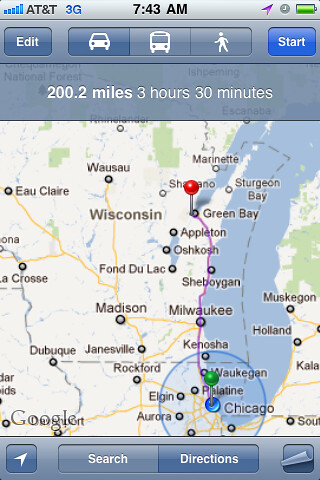This detailed screenshot is from an older model smartphone with AT&T service, displaying a map screen. At the top, on a gray shadowed bar, various status indicators are visible: a blue battery signal suggesting full charge, the text "AT&T" in black, and a "3G" network indicator in blue. The middle of this bar shows the time as "7:43 a.m." in black, and there are additional symbols on the right, including a battery icon. Below this, a grayish-blue navigation bar features buttons for toggling between a white car symbol, a white bus symbol, and a white stick figure symbol, with "edit" on the left and "start" on the right. The main segment of the screen displays a map with cities near Wisconsin, including Milwaukee, Oshkosh, and Kenosha. Above the map, travel details are provided: "200.2 miles, 3 hours, 3 minutes." Numerous blue and gray buttons are present throughout the interface, including search and directions options, indicating that directions have been inputted. The phone is actively trying to locate a position, as suggested by an arrow pointing to the top right.